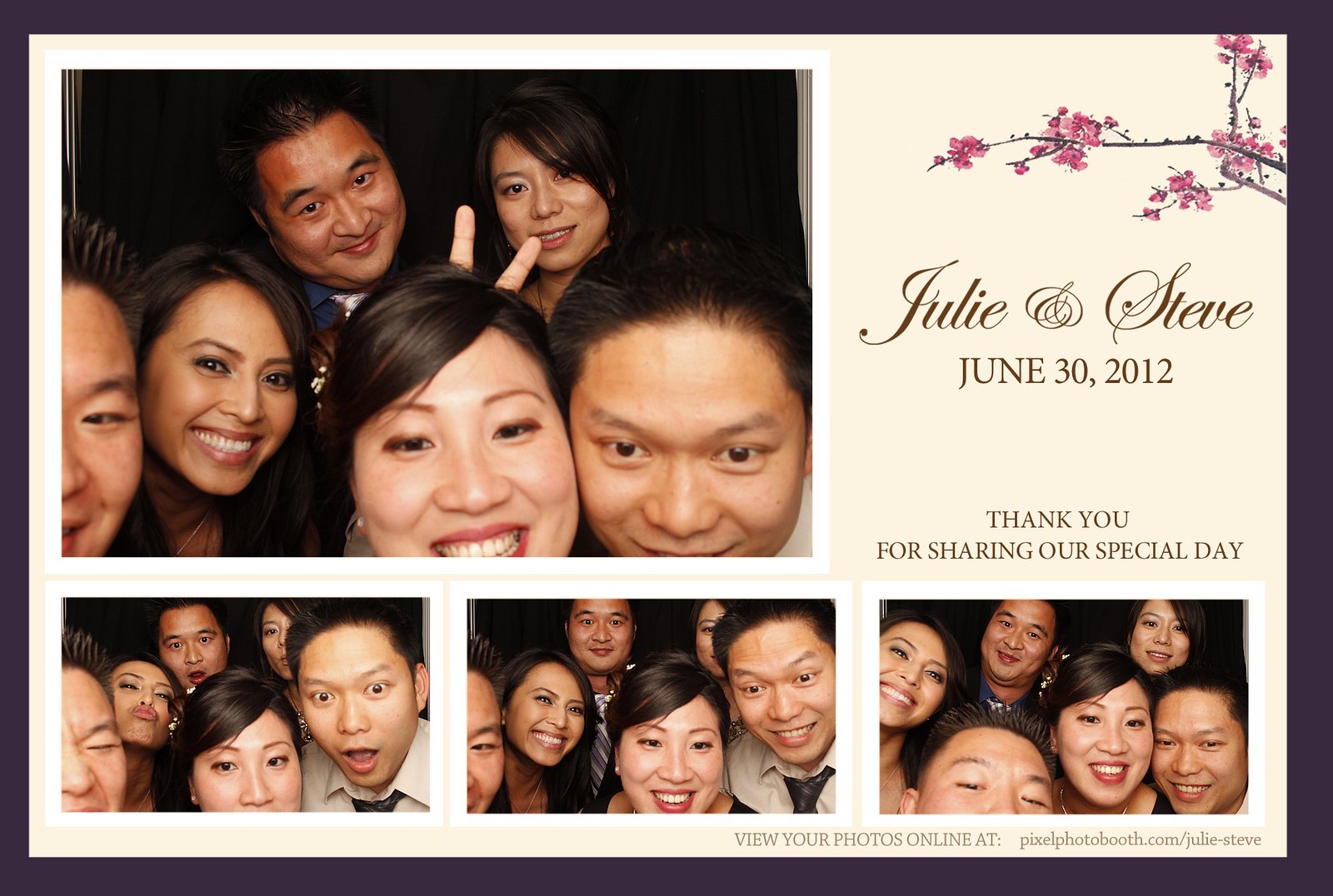The card has a dark purple border and features a collage of four images, all taken at what seems to be Julie and Steve's wedding on June 30th, 2012. The largest photo, displayed in the top left quadrant, shows six people posing together. The bottom row consists of a man, a woman, another woman, and another man, with a man and a woman making a peace sign positioned behind them. Three smaller images beneath the main photo showcase the same group of people in various poses and expressions, enjoying themselves and smiling for the camera. The top right of the card includes text in cursive gray letters that reads, "Julie and Steve," followed by "June 30th, 2012," and "Thank you for sharing our special day" in all capital letters. A decorative element, resembling purple orchid flowers or a cherry blossom branch, adorns this section. At the bottom right, it reads, "View your photos online at pixelphotobooth.com/Julie-Steve," providing a link for guests to access and potentially purchase the photos taken at the event.